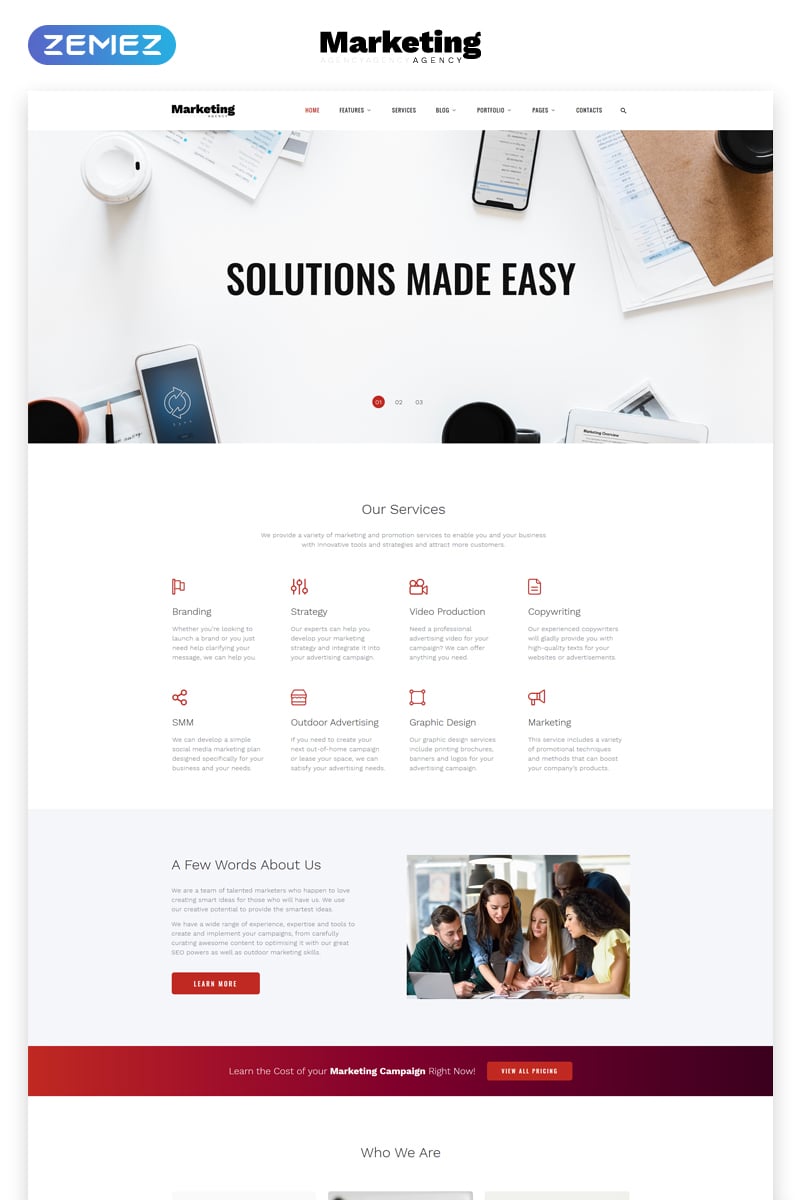In this detailed screenshot of a marketing agency's website, various elements are meticulously laid out, starting with the header. At the very top middle, the prominent black text "Marketing" is displayed, indicating the focus of the website, with a smaller, light gray text below that seems to spell out the word "agency." To the far left of this logo, a distinct oval icon is positioned in the upper left corner, featuring a gradient that transitions from a deep blue to a lighter turquoise. This icon has the abbreviation "Z-E-M-E-Z" in white, capital letters at its center.

Beneath the header lies the website's navigation bar, set within a white border. To the left of the bar is another logo similar to the one above, while the right side hosts the navigation menu. This menu includes options such as "Home" and approximately six other selections in black text. The visibility of these options is hindered by the small and slightly blurry text. Moreover, a magnifying glass icon for search functionality is located on the far right of the navigation bar.

The main background image showcases a white desk adorned with various items, including smartphones, a coffee cup, and scattered papers. Central to this image is the bold black text "Solutions Made Easy." Below this content, a white block is found, highlighting the header "Our Services" in black, followed by a brief, albeit unreadable, description.

Displayed within this section are eight service categories, each accompanied by distinct red icons and brief descriptions. The first row features a red flag icon labeled "Branding," a red dials icon denoted "Strategy," a red camera icon for "Video Production," and a red document icon for "Copywriting." In the subsequent row, icons include a connection diagram marked "SMM," a hamburger-like symbol titled "Outdoor Advertising," a red square with circles at the corners for "Graphic Design," and a megaphone icon designated as "Marketing."

Directly beneath this white service block is a light gray section. Positioned slightly off-center to the left, a header reads "A Few Words About Us," followed by two small, unreadable paragraphs. A prominent red rectangular button, stating "Learn More" in white text, lies beneath these paragraphs. To its right, there's an image capturing office employees collaborating at a desk. This picture includes a white man seated, two white women, a standing black man, and a mixed-race woman with curly hair all engaged in discussion.

Further down, a thin, gradient block extends horizontally, transitioning from red on the left to dark purple on the right. In white, the text reads "Learn the cost of your marketing campaign right now," with "marketing campaign" in bold. Adjacent to this text is a blurry red button, possibly indicating "View All Prices."

Finally, a white block beneath this gradient section has a heading that says "Who We Are" in black. Visible within this block is the top portion of three boxes, potentially indicating photos or additional content, hinting at more information further down the page which is not shown in the screenshot.